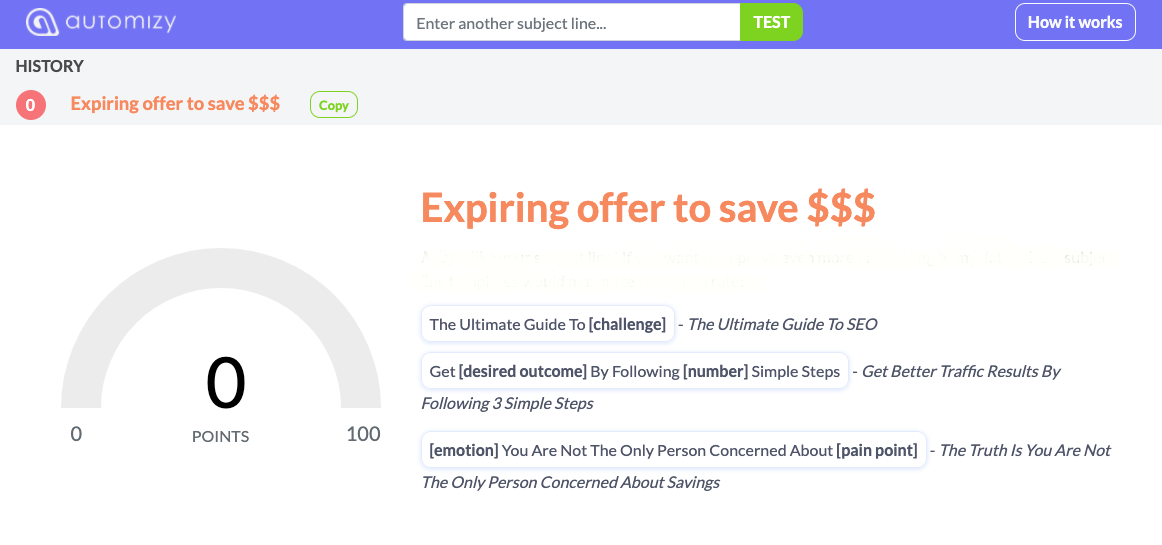The top ribbon of the website features the logo "AUTOMIZY" prominently displayed. Below this, there is an input box prompting users to "Enter Another Subject Line," accompanied by a green "Test" button to its right. On the far right side of the page, there is a link labeled "How It Works."

Underneath the AUTOMIZY header, a gray informational box can be seen, displaying "History" alongside a red circle containing a zero. The text within the box reads, "Expiring Offer to Save $$$," with a "Copy" button positioned beside it.

The main section of the page, which is predominantly white, houses a dashboard on the left featuring a half-circle gauge ranging from 0 to 100. Currently, the gauge points to zero, and in the center, it states "0 Points." Above this in orange text, the phrase "Expiring Offer to Save $$$" appears once again.

Within this primary area, there is a prominent button titled "The Ultimate Guide to (Challenge)," followed by text stating "The Ultimate Guide to SEO" outside of its containing box. Adjacent to this, another box includes the text, "Get (Desired Outcome) by Following (Number) Simple Steps," with the associated message, "Get Better Traffic Results by Following Three Simple Steps," displayed outside the box.

Further down, another boxed section reads, "(Emotion) You Are Not the Only Person Concerned About (Pain Point)," with a follow-up statement outside the box reading, "The Truth is You Are Not the Only Person Concerned About Savings."